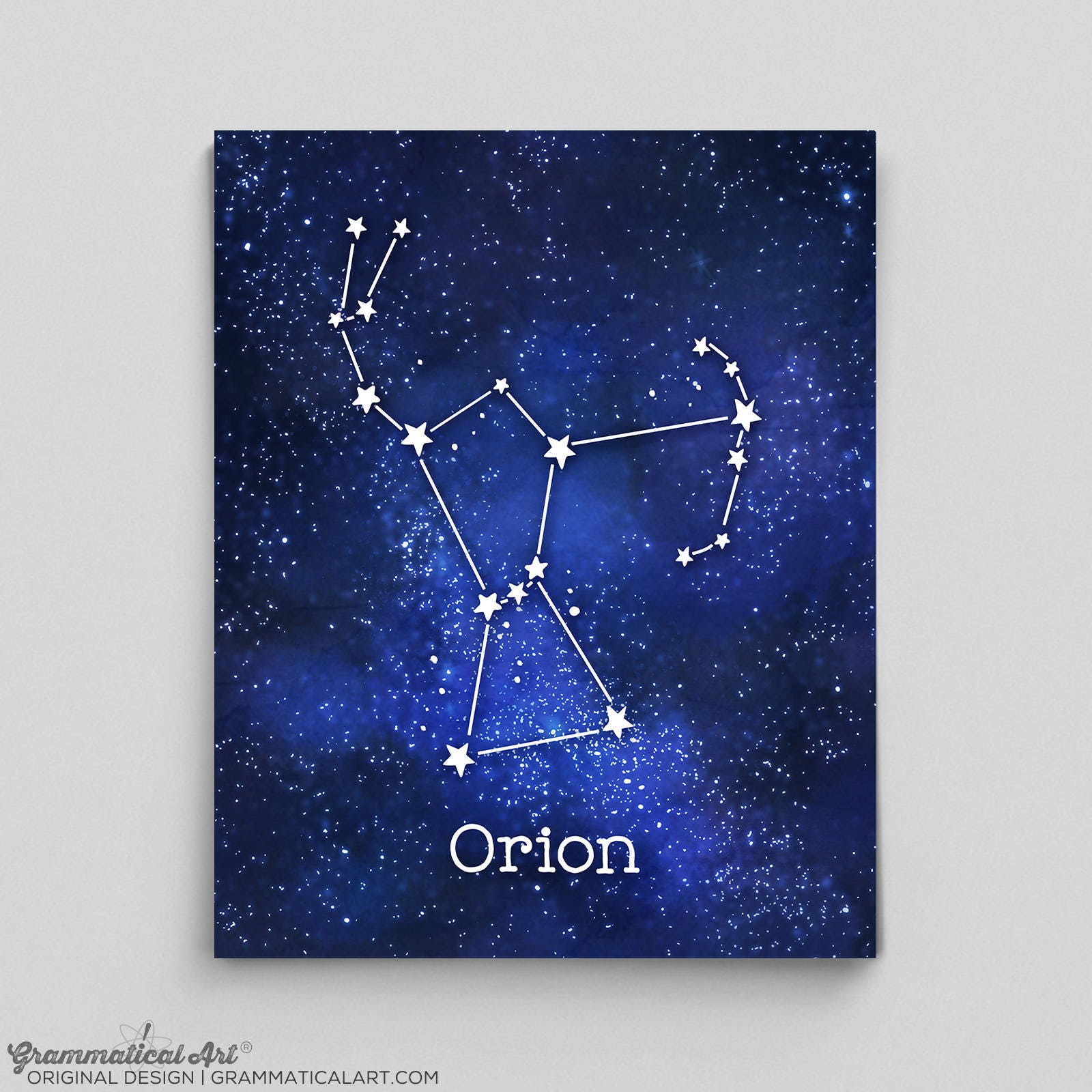This digital artwork depicts the constellation Orion set against a varying dark and lighter blue background, emulating a starlit night sky. The piece shows a celestial scene dotted with numerous white stars, each represented by the classic five-pointed star shape in various sizes. The stars of the Orion constellation are prominently connected by white lines, vividly forming the figure of the mythological hunter, Orion. His right arm is depicted raised behind him, holding an arrow, while his left arm stretches forward, grasping a bow. The signature features, including Orion's belt, composed of three stars aligned through the middle, and a trapezoid shape formed by the stars of his lower body, are clearly outlined. Below the constellation, "Orion" is written in white text. The artwork is bounded by a gray border, which includes the inscription "grammatical art, original design, grammaticalart.com" in the bottom left corner, signifying its unique and original creation.